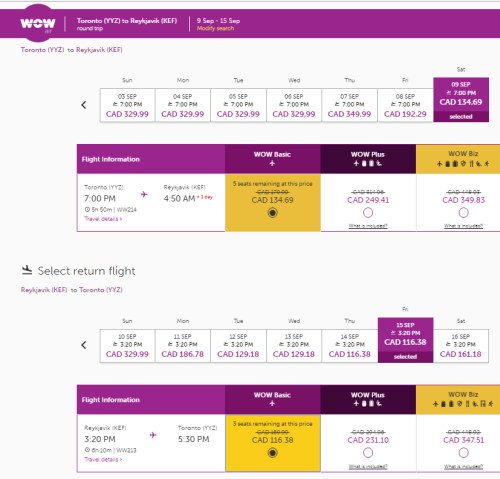The image depicts a website, featuring a clean, white background. At the top of the page, there is a medium purple banner that subtly blends in hints of pink and red. Within this banner, the text reads "What is the line?" accompanied by a circular emblem with white text inside that says "Wow."

Below this banner, the text continues, stating: "Toronto (YYZ) to Reykjavik (KEF)" indicating a round-trip flight from September 9th to September 15th. There is a "Modify Search" option positioned nearby.

Descending further, the website provides a detailed flight schedule under the heading "Toronto to Reykjavik." The dates are sectioned by days of the week: Sunday, Monday, Tuesday, Wednesday, Thursday, Friday, and Saturday. 

- Sunday, September 3rd: CAD $329.99
- Monday, September 4th: CAD $329.99
- Tuesday, September 5th: CAD $329.99
- Wednesday, September 6th: CAD $329.99
- Thursday, September 7th: CAD $349.99
- Friday, September 8th: CAD $192.99
- Saturday, September 9th: CAD $134.69

Following the price chart, the website presents sections labeled "Flight Information" and "Select Return Flight," listing relevant return flight prices.